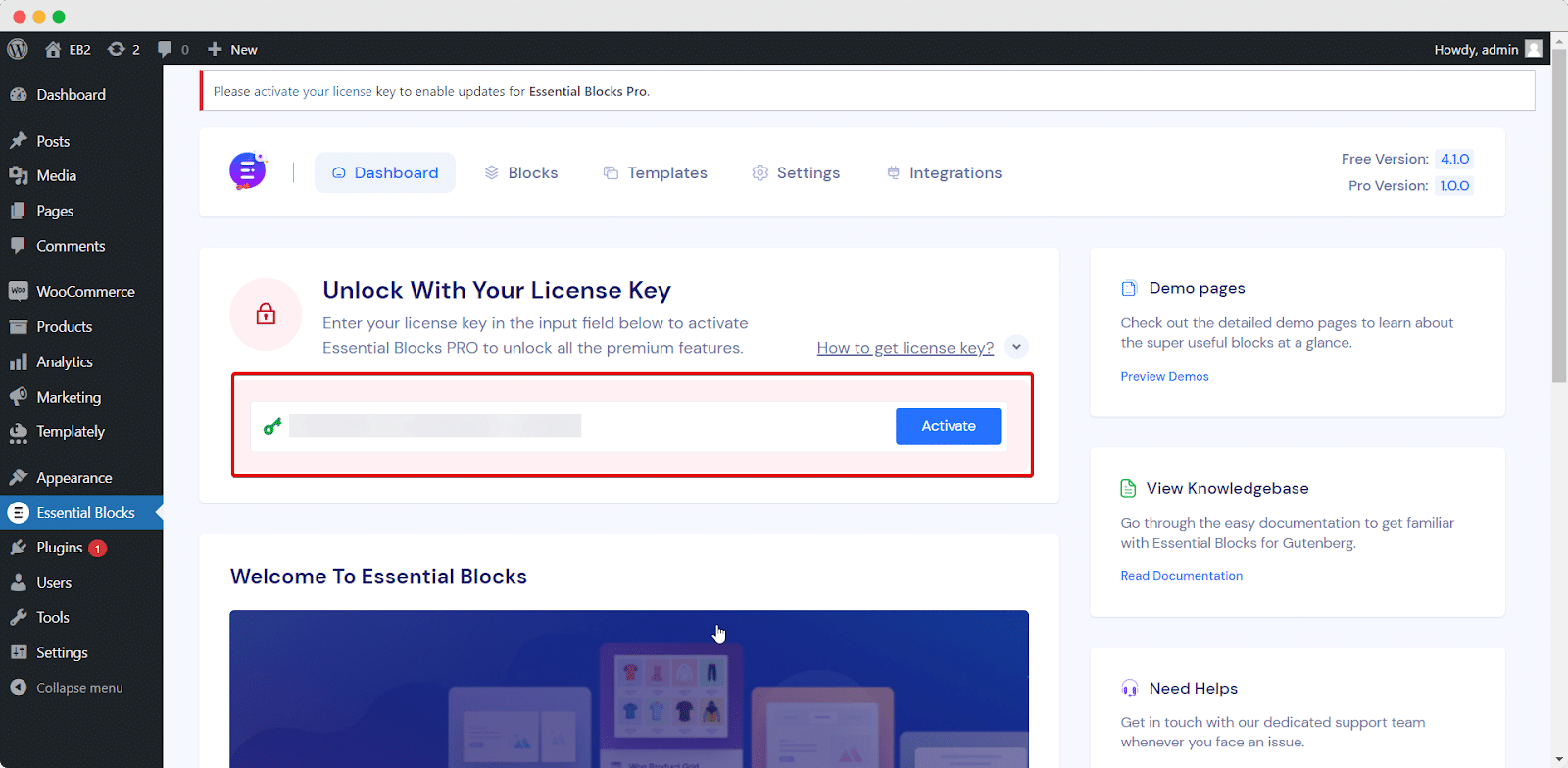This screenshot captures the interface of a website, presumably one related to web design or website management, possibly using WordPress given the distinctive icon visible. 

On the left-hand side encased within a black border, there is a navigational menu adorned with white text. Features listed include:

1. **Dashboard**
2. **Posts**
3. **Media**
4. **Pages**
5. **Comments**
6. **WooCommerce** (stylized as W-O-O commerce)
7. **Products**
8. **Analytics**
9. **Marketing**
10. **Template**
11. **Appearance**
12. **Essential Blocks** (highlighted in blue)
13. **Plugins** (with a notification circle displaying the number 1 in red)
14. **Users**
15. **Tools**
16. **Settings**
17. **Collapse Menu**

Immediately to the right of this menu, in a horizontal header with a black background, a sequence of icons and text links are aligned:

- A **WordPress icon** (W within a circle).
- A **House icon** labeled “EB2”.
- A **Refresh icon** (depicted as circular arrows) marked with the number 2.
- A **Chat icon** indicating zero messages.
- A **Plus icon** adjacent to the word “New”.
- On the far right, there is a greeting saying "Howdy, Admin," accompanied by a blank profile picture icon.

Centrally located on the interface is a prominent rectangular box with the following details:

- **Message**: “Please activate your license key to enable updates for Essential Blocks Pro.”
- **Headings** underlined for orderly navigation: **Dashboard**, **Blocks**, **Templates**, **Settings**, and **Integrations**.
- An **information block** on the right side indicating the software versions: “Free version 4.1.0, Pro version 1.0.0.”

Beneath this is a section titled “Unlock with your license key”. Here, users are prompted to input their license key in a designated field and then click a blue button labeled “Activate” to proceed.

This organized layout emphasizes ease of navigation and straightforward access to key functionalities and administrative options essential for managing a WordPress-based site.